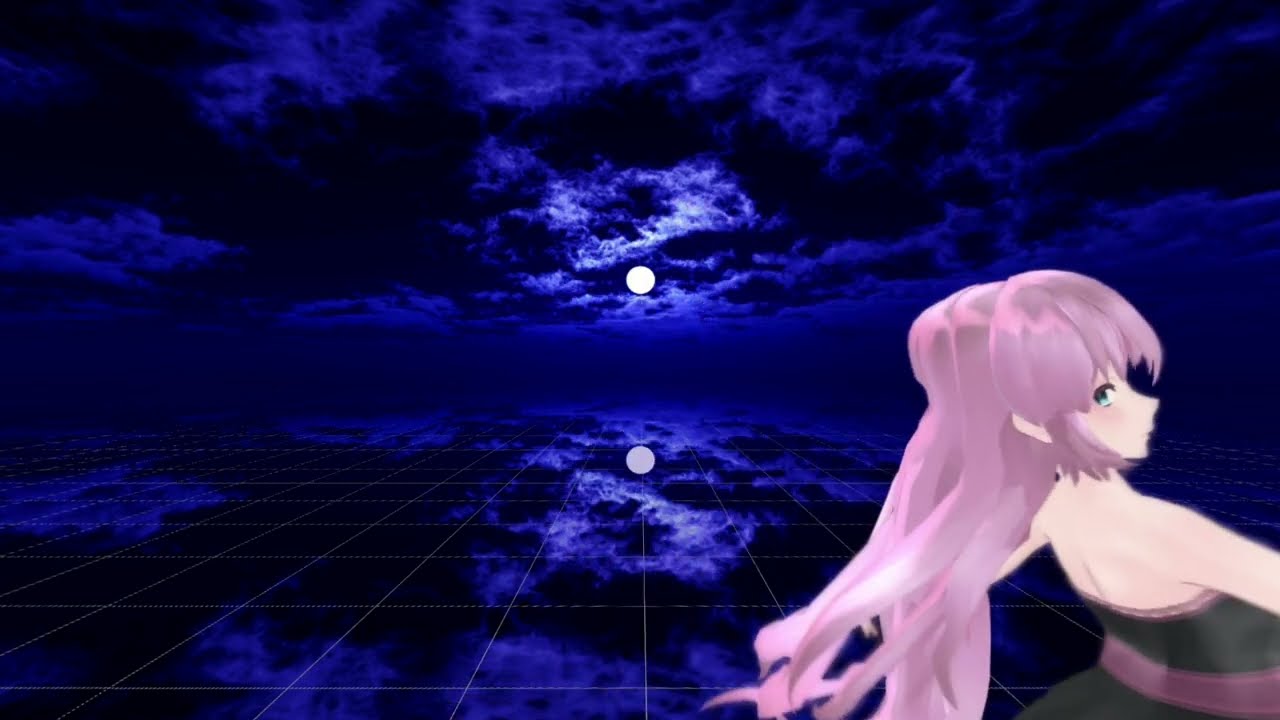This digital art image features a captivating scene with a large reflective glass floor composed of square tiles. Above, the sky transitions through various shades of blue, from bright to nearly black, and is adorned with a luminous white moon at its center. The celestial display, including dark and blue-tinted clouds, is vividly mirrored on the glass surface below, enhancing the ethereal atmosphere.

In the bottom right corner stands an anime girl with flowing, light pink hair cascading past her shoulders. She has delicate, white skin and large, expressive blue eyes. The girl is clothed in a sleeveless, shoulderless black and pink dress, complemented by a soft pink belt at the waist. She stands gracefully on the reflective grid, adding a dynamic contrast to the geometric, perspective-driven background that fades into the distance.

The overall composition, with its intricate reflection and rich variation in color, creates a surreal and dreamy visual experience.